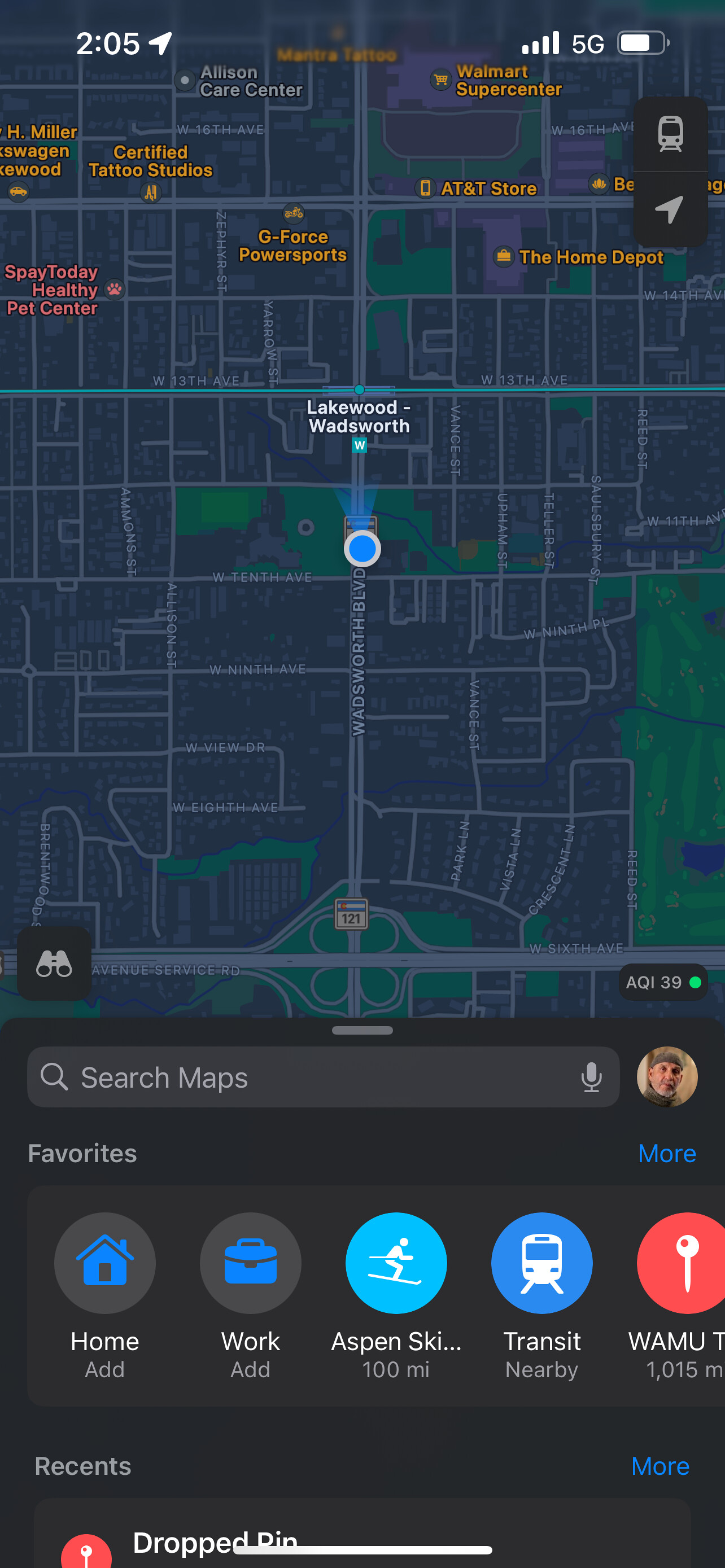Displayed on a smartphone screen is a detailed map interface. At the top-left corner, a white arrow points towards the upper-right corner next to the text "2.05." To the right, the phone's status bar shows four bars of signal strength, a "5G" label in white, and a battery icon that is predominantly white with a gray section indicating a partially drained charge.

The map itself is a blue-gray canvas with lighter gray lines denoting streets, such as Wadsworth Boulevard. Notable businesses are marked with gray circular icons and labeled in orange text, including AT&T Store, The Home Depot, Walmart Supercenter, Certified Tattoo Studios, and GeForce Power Sports. Patches of green suggest areas of vegetation, possibly woods or forests.

At the bottom of the screen, a dark gray rectangular search bar contains the text "Search map." To the right of this bar, there is a small profile picture of an older Indian man with a white beard, wearing a gray hat and a gray turtleneck. Below the search bar, blue text reads "More," followed by circular quick-access icons labeled "Home," "Work," "Aspen Ski 100 miles," and "Transit Nearby." Additional text items are partially visible, including "WAMU," and a truncated label starting with "T" and ending with "1015M."